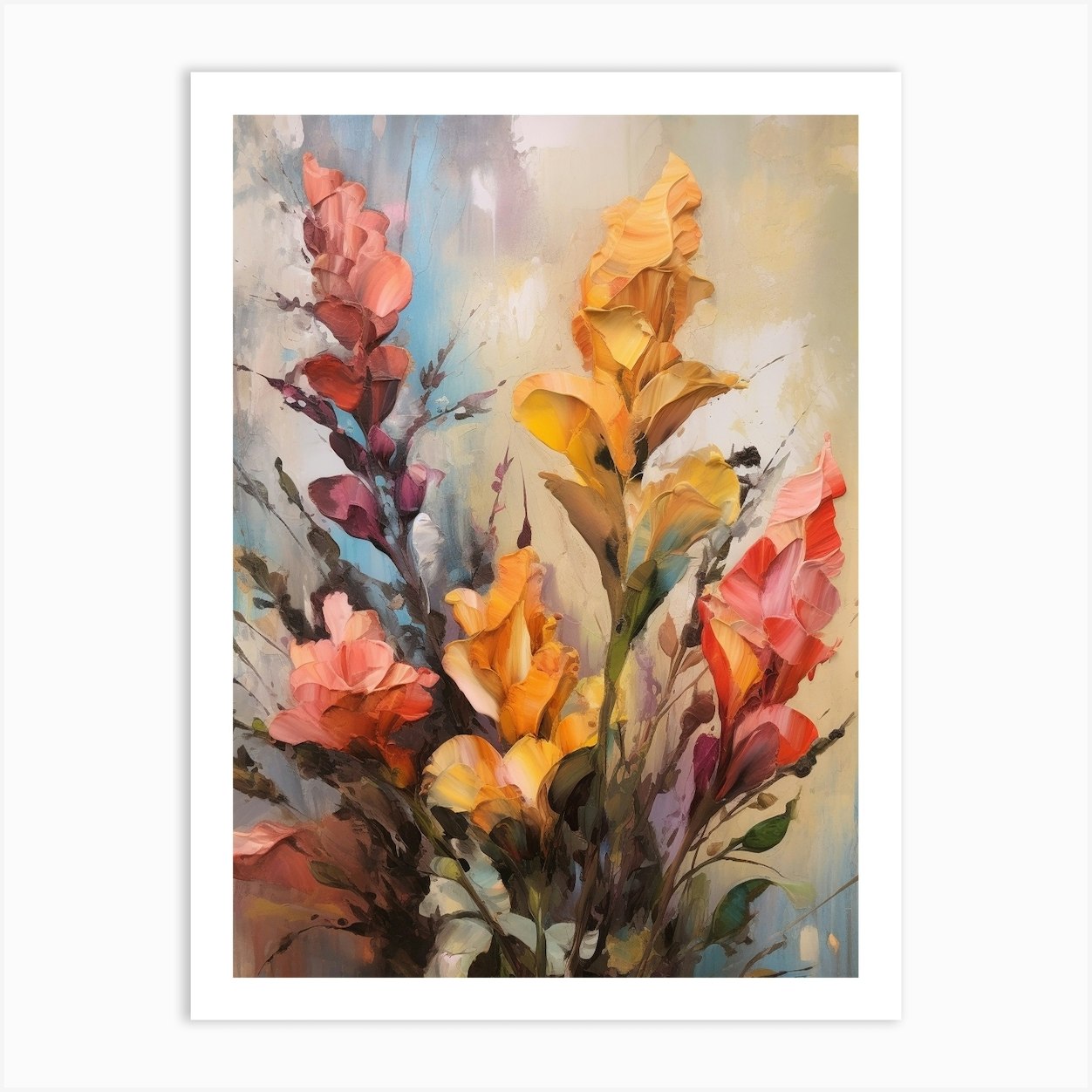This close-up photograph captures a detailed and professionally presented painting of flowers, framed within a white picture frame that hangs against a plain white wall. The artwork, which resembles a watercolor piece with an abstract touch, features a white background on what seems to be a portrait-oriented canvas. The backdrop of the painting showcases a blend of light yellow, bluish-gray, green, brown, and white hues, resembling a sky with light blue clouds.

Centered around the canvas are an array of flowers, primarily depicted with a sense of fluidity and artistic smudge. Positioned towards the top left is a light pinkish flower, while a yellow flower occupies the right portion and an orange flower is situated in the middle underneath these. Each flower features long stems and green leaves reaching up from the bottom of the artwork. The color palette of the flowers also includes nuances of peach-orange and hints of purple and white, contributing to the vibrant yet enigmatic composition of the piece. This painting, whether a renowned work or an evocative abstract floral study, conveys a rich artistic depth through its use of color and form.